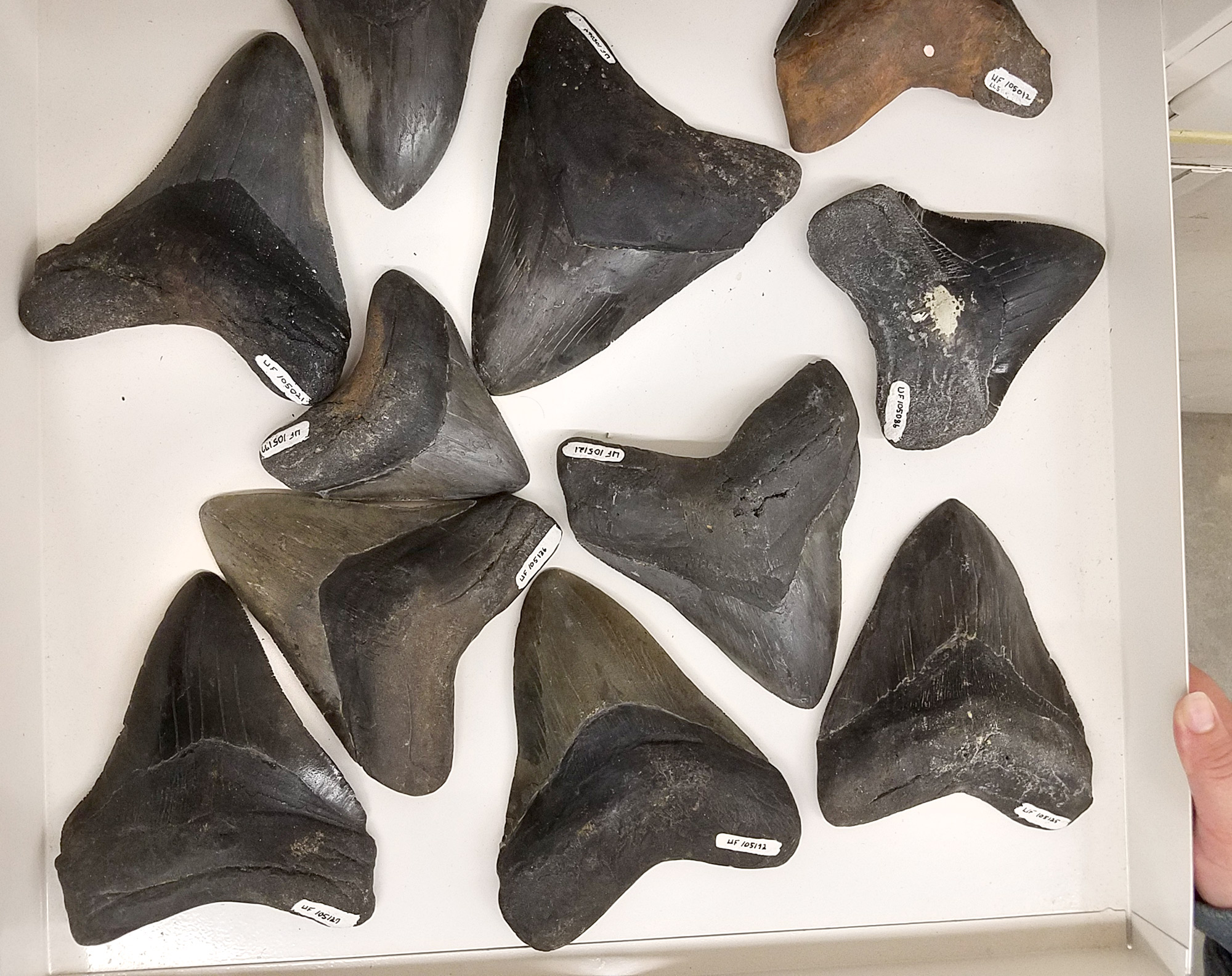In the image, there is a white box held by a person's thumb and pointer finger on the bottom right corner. The box appears to be oriented either flat, looking down on it, or possibly displayed on a wall, as it contains heavy objects that wouldn't stay in midair without support. Inside the box, there are 11 large specimens that resemble fossilized shark teeth. These teeth are enormous, much larger than the hand holding the box, indicating that they came from gigantic creatures. The teeth are predominantly black or dark gray with some tan and white pieces, and each one is labeled with small white labels that have black writing, though the text is hard to discern. The teeth have a conical top that narrows, becoming thicker towards the bottom, forming an almost triangular shape with a slight curve at the base. The overall appearance suggests that these could be part of a museum collection or some scientific display, showcasing an impressive and ancient discovery.